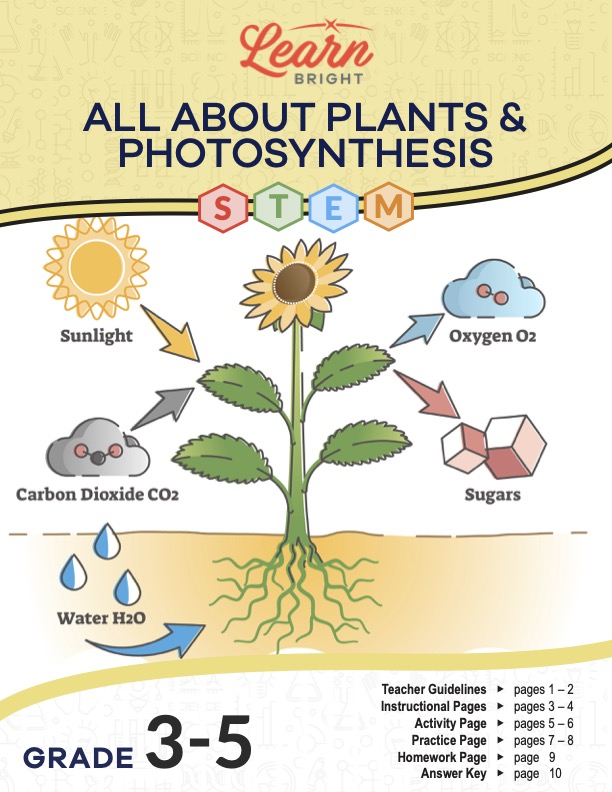The image is a vibrant, portrait-oriented cover of a science book, "Lean Bright," designed for students in grades 3 to 5. The top of the page features the company's logo, with "Lean" in fancy red cursive text, "Bright" in smaller grey brick text, and a line with an X in the middle, forming the complete logo. Below the logo, in a playful, multi-colored hexagon pattern, is "All About Plants and Photosynthesis," emphasizing STEM education with a red S, green T, blue E, and orange M.

The main illustration showcases the process of photosynthesis with a detailed and colorful diagram of a sunflower. Sunlight, represented by an image of the sun, arrowed towards the sunflower, highlights the energy inputs. Carbon dioxide, depicted as a cloud with pink circles labeled CO2, points towards the leaves. The roots absorb water, shown as blue drops labeled H2O, with arrows indicating the flow into the plant. The plant then releases oxygen, illustrated by a cloud with double pink circles labeled O2, and produces sugars, represented by small pink sugar cubes.

The bottom of the page lists the book's contents, detailed in black text: "Grade 3 to 5" on the left and a comprehensive index on the right. The index includes "Teacher Guidelines: pages 1-2," "Instructional Pages: pages 3-4," "Activity Page: pages 5-6," "Practice Page: pages 7-8," "Homework Page: page 9," and "Answer Key: page 10," all marked with black triangles pointing to the corresponding pages. The background features light yellow and blue stripes, adding to the engaging and educational aesthetic.